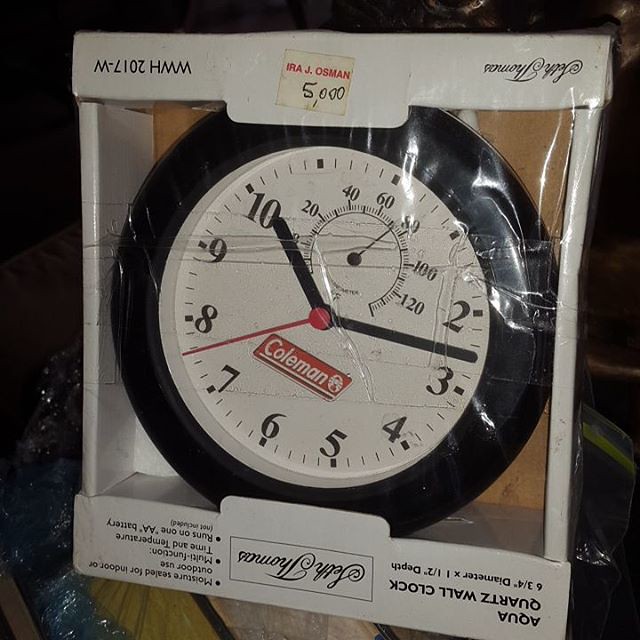This image features a wall clock still inside its packaging, though the packaging appears to have been resealed. The clock itself has a round black edge and a white face, with black hour and minute hands, and a red second hand. It is marked with the numbers 10 and 12, indicating its design for easy reading. Notably, there is an additional gauge at the center of the clock face that displays temperature, currently indicating 71 degrees Fahrenheit, with a range extending from below zero to 130 degrees.

The clock is branded as Coleman, but the packaging, which is upside down and secured with clear tape over cellophane, is labeled Seth Thomas Aqua Quartz Wall Clock, suggesting a mismatch between the product and its packaging. A price tag on the packaging reads "Ira J. Osman 5000." The background of the image shows some packing materials, indicating the clock might have been recently taken out of a larger box.